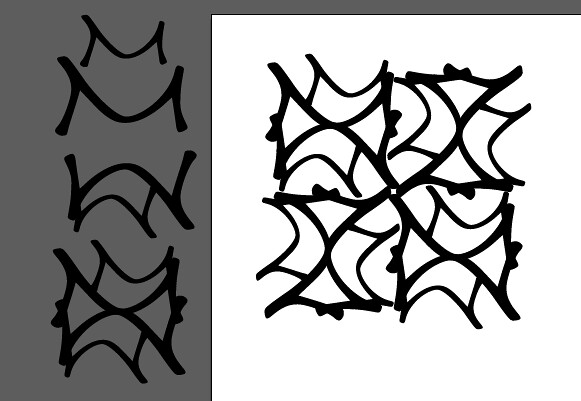This detailed image features an array of intricate designs, predominantly rendered in grayscale. The composition includes two main color schemes: gray and black, and white and black, offering a stark contrast that enhances the visual interest. The objects within the design are positioned adjacent to each other, forming cohesive groups. Some elements are arranged vertically from top to bottom, while others are centrally clustered, creating a complex yet organized pattern. The artwork, which could either be computer-generated or meticulously hand-drawn and then digitized, showcases a blend of artistic precision and creativity. The meticulous detailing in the designs suggests a high level of craftsmanship, making it a striking piece whether viewed as a digital rendering or a traditional print.